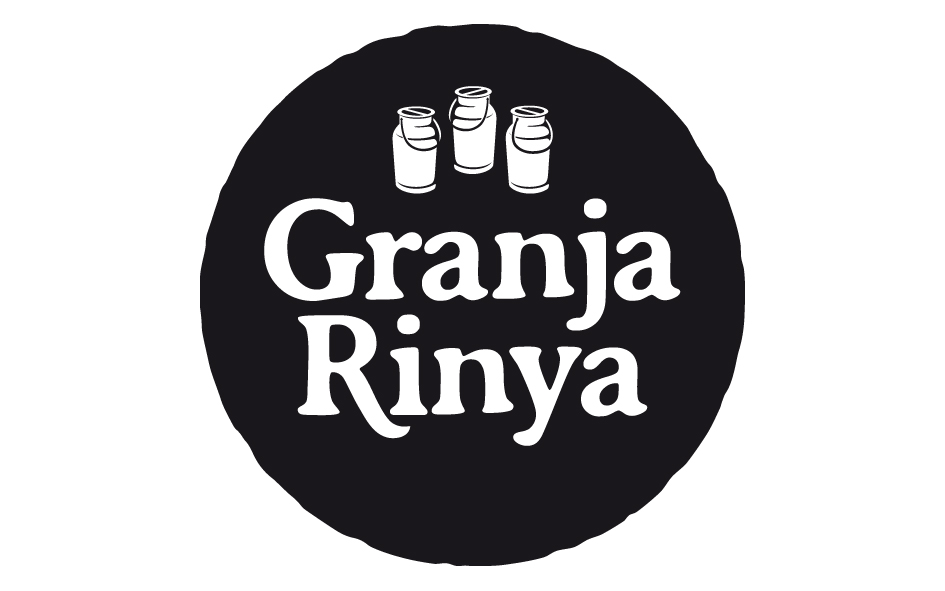The image is a black circle with slightly rough borders, featuring a white serif font that reads "Granja Rinya" in bold. The word "Granja" is positioned above "Rinya" at the center of the circle. Above the text, there are three small, old-school milk jugs, each with a round cap and a black handle hanging down, suggesting they might contain milk. The logo is purely black and white, with no other colors or contextual elements.